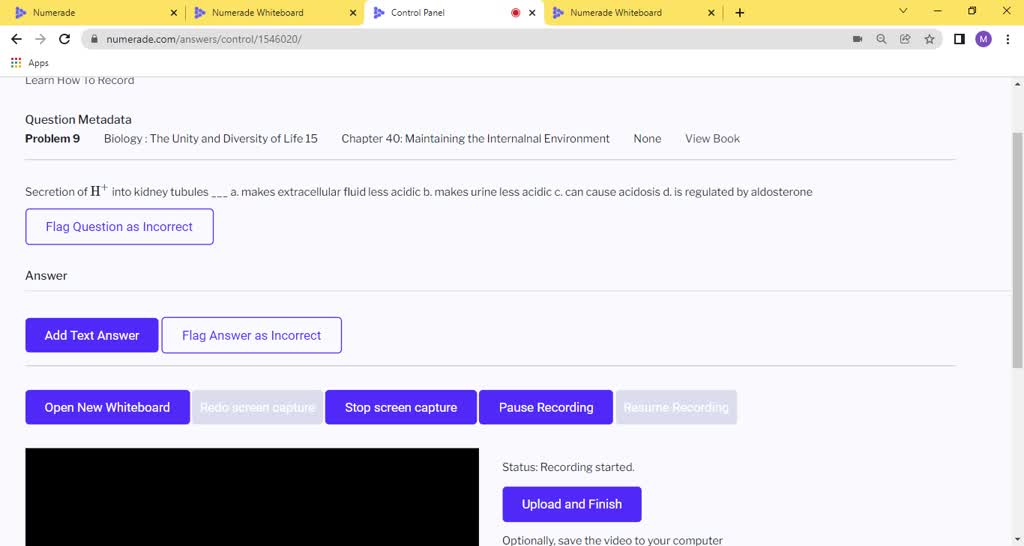This screenshot depicts the interface of the Numerade website, identified with a logo comprising six purple dots arranged in a triangular formation resembling a play button. The screenshot displays multiple browser tabs, including the website's Home tab, two Whiteboard tabs, and a Control Panel tab, all highlighted in yellow, except the Control Panel tab, which is in white.

Prominently featured at the top is the URL field, accompanied by user interface icons: an "M" representing the user's profile, and a grid symbol for applications. Directly underneath, there are options related to recording on the site, notably the prompt to "Learn How to Record."

The Control Panel focuses on question metadata for "Problem 9" in the "Biology of the Unit and Diversity of Life" section from Chapter 40 titled "Maintaining the Internal Environment." The specific question discussed involves the secretion of H+ in kidney tubules, offering multiple-choice options:

- A) Makes extracellular fluid less acidic
- B) Makes urine less acidic
- C) Can cause acidosis
- D) Is regulated by aldosterone

A flagged indication marks the answer as incorrect. The Control Panel also presents options in purple for interacting with recordings, including "Open Your Whiteboard," "Stop Screen Capture," and "Pause Recording." Two grayed-out options are illegible, followed by the status indicator "Recording Started" and the final options to "Upload and Finish."

This interface section offers tools for users to record, manage, and upload educational content, reflecting Numerade's focus on facilitating online learning and instructional videos.